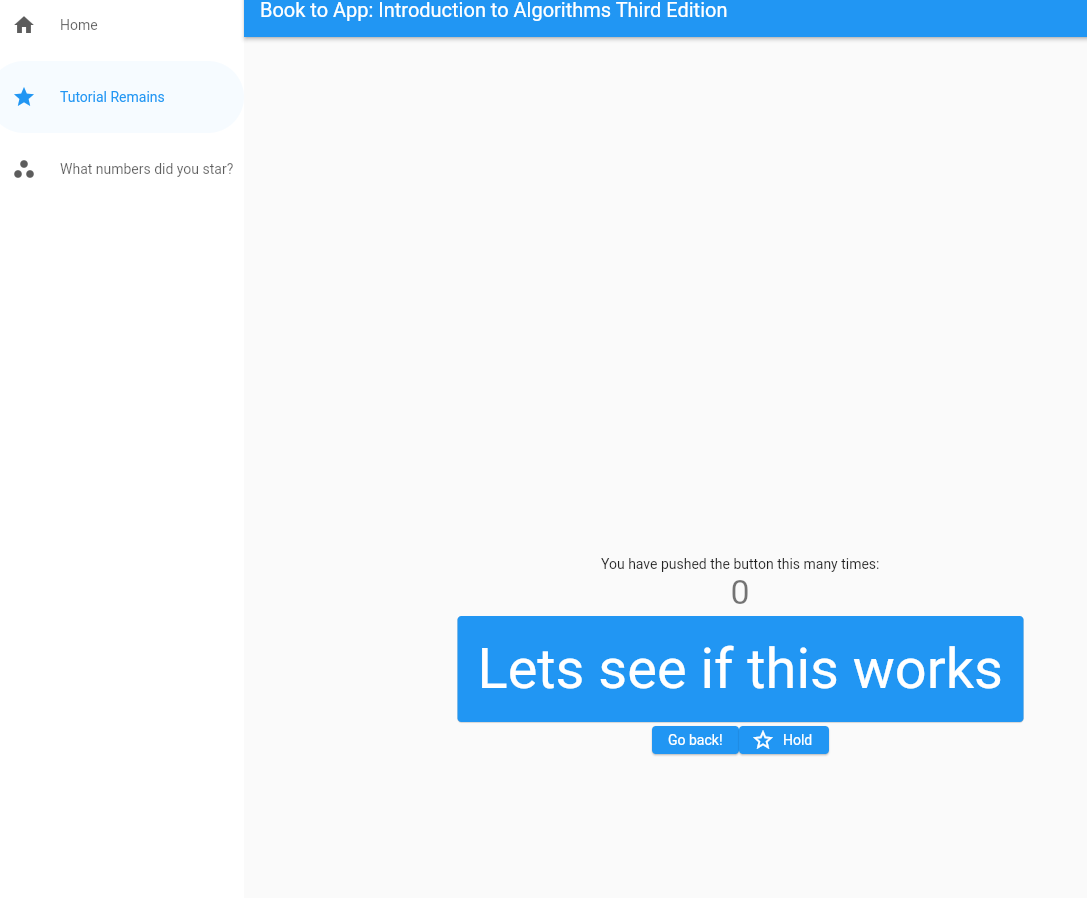The image depicts a tutorial web page with a blue header at the top displaying white text that reads, "Book to App: Introduction to Algorithms, Third Edition." On the right side of the header, there is a white section containing a home icon and the text "Home," a star icon with text that reads "Tutorial Remains" — which is highlighted in blue, and a triangle icon followed by an ellipsis and the phrase "What Numbers Did You Star."

The main body of the web page has a light gray background. Black text on this background states, "You have pushed the button this many times," with the number "0" displayed beneath it. Below this, there is a blue box containing white text that reads, "Let's see if this works." Further down, there are two smaller buttons both with white text on them: the left button says "Go Back!" and the right button, which features a star icon, reads "Hold."

To summarize, the web page header includes "Book to App: Introduction to Algorithms, Third Edition" with navigation tabs for "Home," "Tutorial Remains" highlighted in blue, and "What Numbers Did You Star." The content area provides feedback on button clicks and includes interactive elements for user interaction.